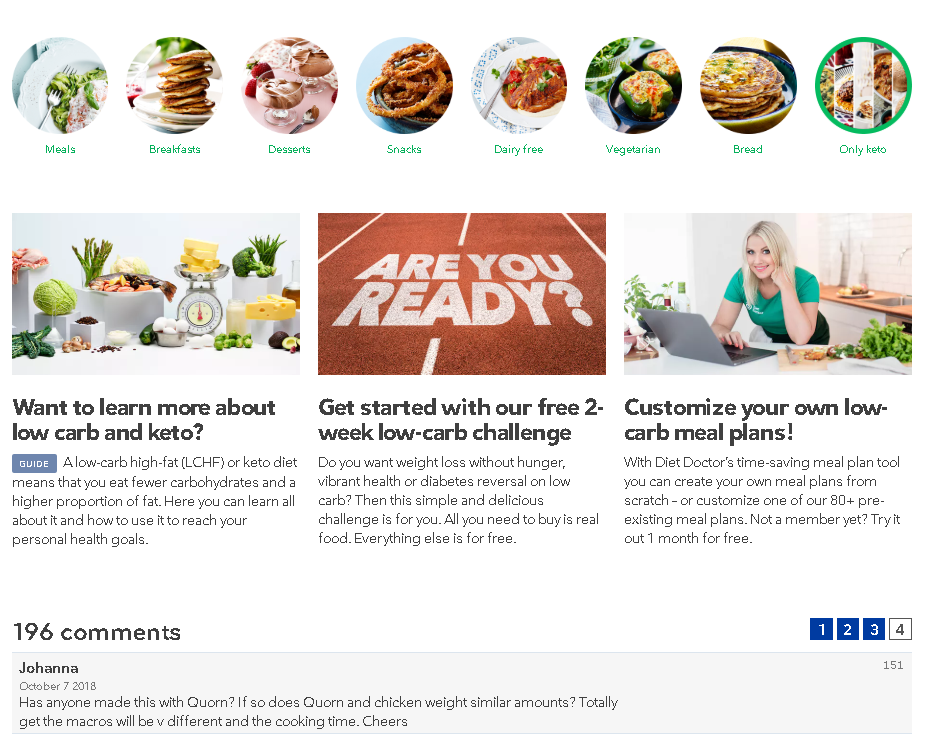The image showcases various diet plans and meal options for individuals interested in low-carb and keto diets. It features three prominent sections, each with a detailed description underneath:

1. **Exploring Low Carb and Keto Diets**: The first section invites users to learn more about low-carb and keto diets, providing a guide for in-depth information.

2. **Two-Week Low Carb Challenge**: The second section encourages users to embark on a free two-week low-carb challenge, with a call to action, "Are you ready? Get started."

3. **Customizable Low Carb Meal Plans**: The third section offers customizable low-carb meal plans with a one-month free trial, urging users to "Try it out."

Above these sections, there is a menu with eight categories to refine meal choices:
- Meals
- Breakfast
- Desserts
- Snacks
- Dairy-Free
- Vegetarian
- Bread
- Only Keto

This allows users to narrow down their preferences and focus on specific dietary needs.

Additionally, the image includes a snapshot of community engagement, showcasing comments from users. One highlighted comment from Johanna, dated October 7th, 2018, inquires about using Quorn (a meat substitute) in meal plans, specifically comparing it to chicken in weight and usage.

Overall, the image serves as a comprehensive guide to low-carb and keto dieting, complete with plans, customization options, and community feedback.